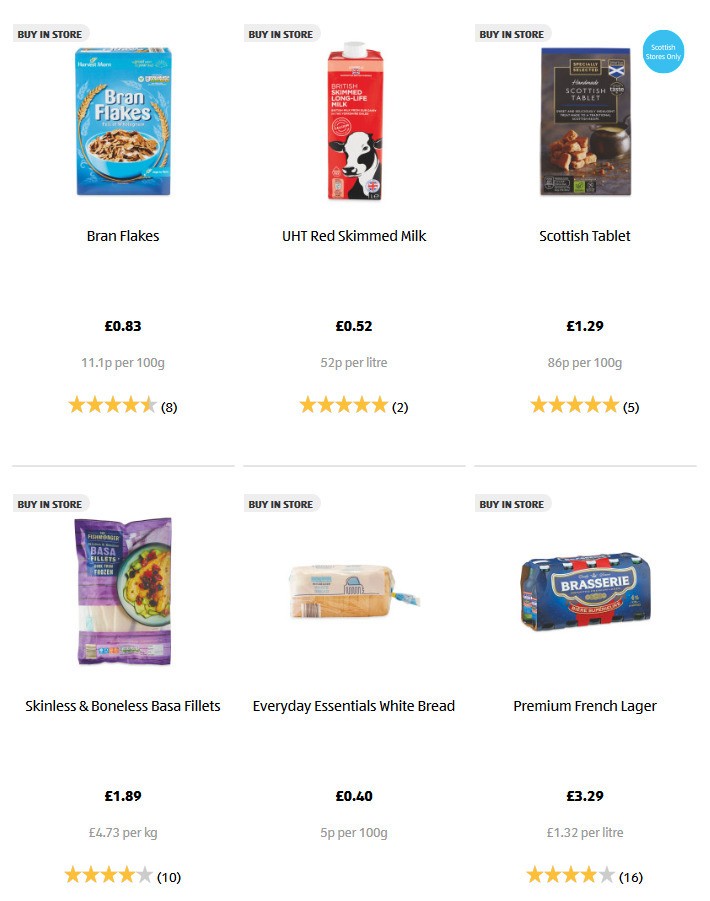A screenshot of an e-commerce website showcasing a selection of various products arranged in two rows, each containing three items. 

In the top row:
1. Bran flakes priced at $0.83.
2. Red-skinned milk priced at $0.52.
3. Scottish Tablets priced at $1.29.

In the bottom row:
1. Skinless and boneless pasta fillets priced at $1.89.
2. Everyday Essentials white bread priced at $0.40.
3. Premium French vodka beer priced at $3.29.

Each product is clearly displayed with its corresponding price, offering a glimpse into the diverse range of items available for purchase on the website.